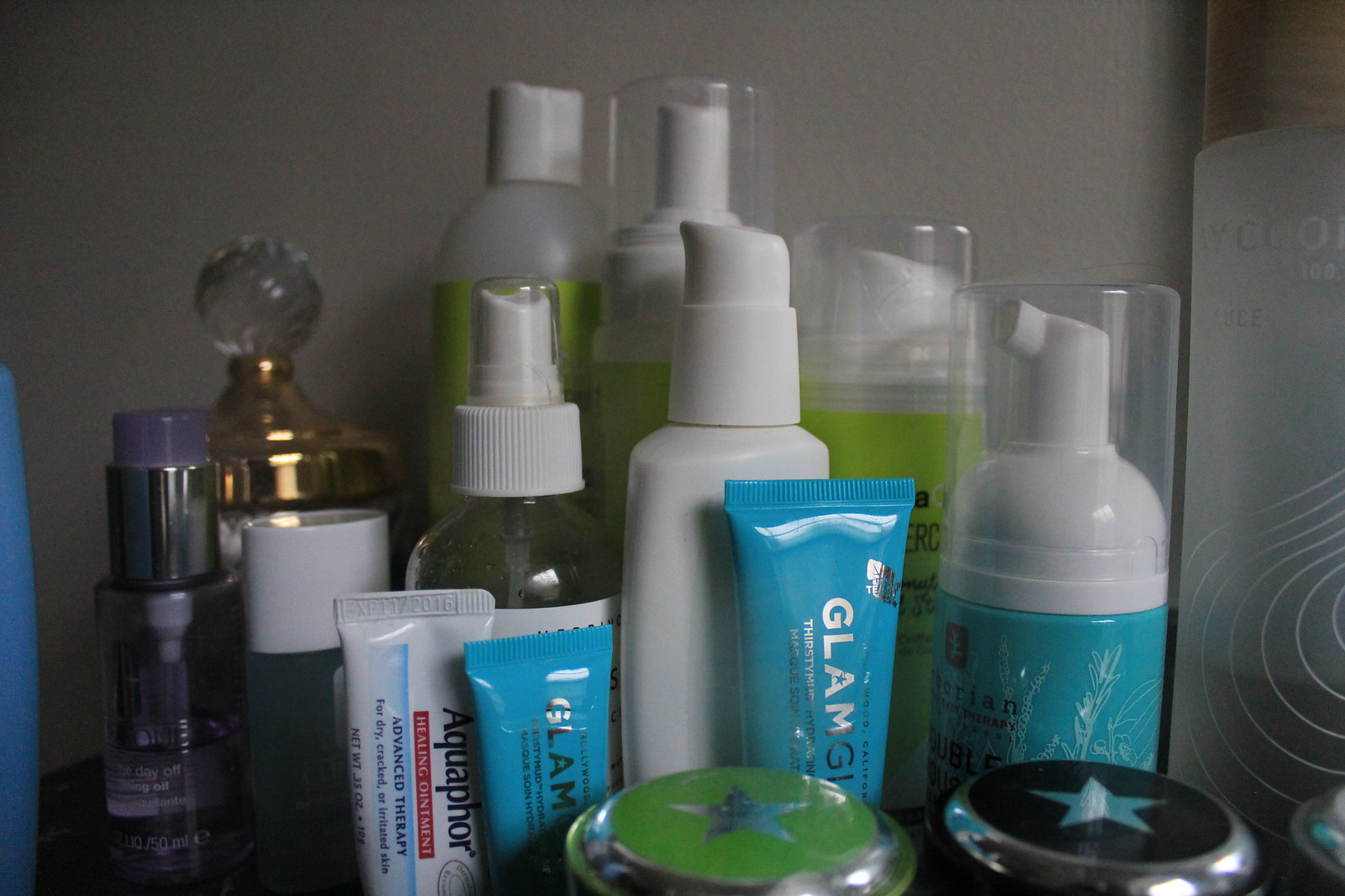The image captures an assortment of personal care products meticulously arranged on a bathroom counter. At the back, a crystal-topped perfume bottle with a gold lid stands elegantly. Beside it, a smaller, purple-hued perfume bottle adds a splash of color. Dominating the scene are various sized tubes and pump bottles, one of which likely dispenses face soap. A distinctive Aquaphor container, recognizable by its advanced therapy lotion label, suggests its use for lip care.

In the foreground, two circular compacts with lids adorned with silver stars—one green, the other black—perhaps contain makeup or powder. Teal tubes marked "Glamour Girl" in two different sizes are prominently displayed. On the far right, a coordinated set with green labels appears to include a shampoo, conditioner, and possibly a detangling spray. This well-organized collection of toiletries reflects the essentials for daily grooming routines.